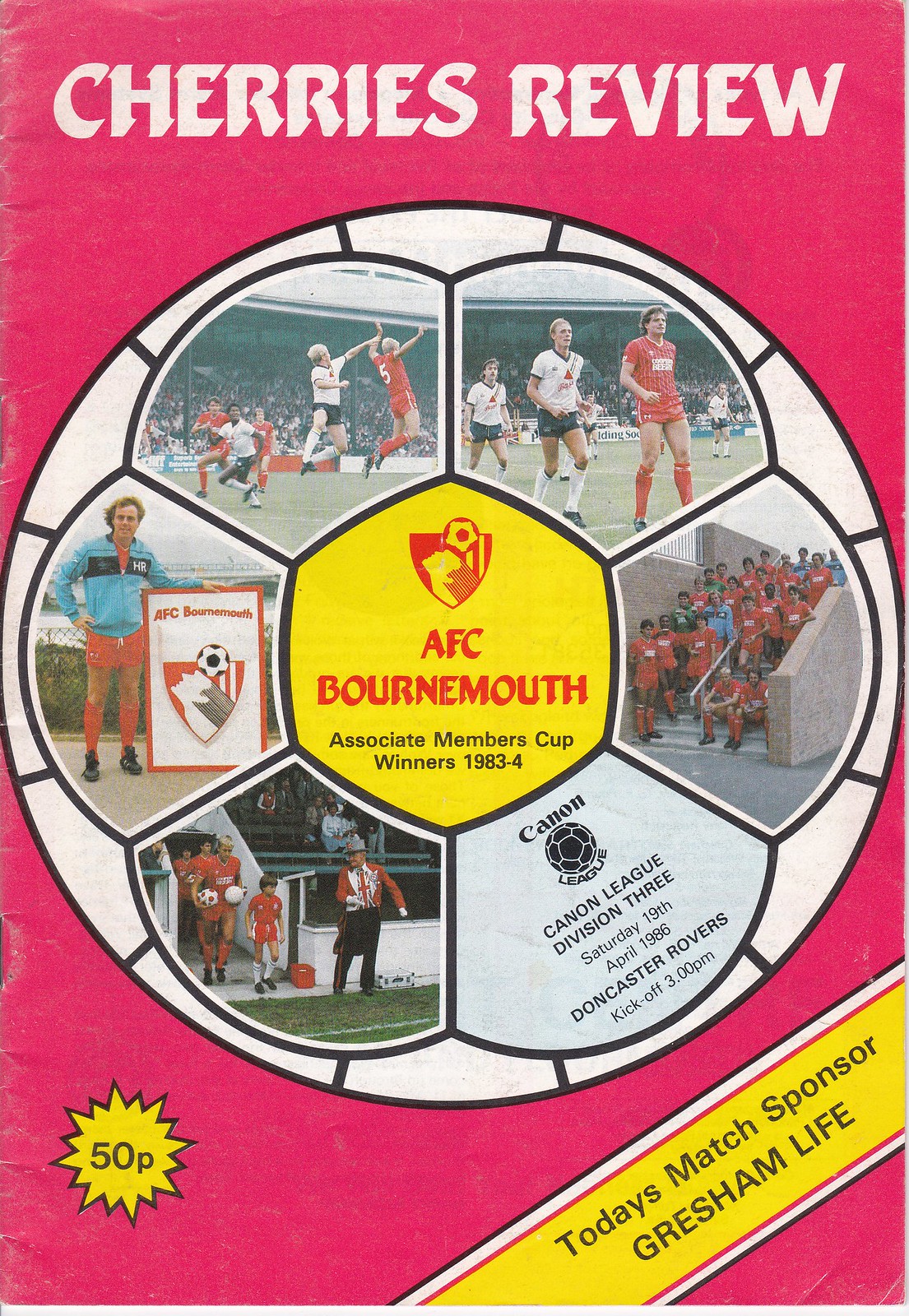The image is a highly detailed cover of a football program titled "Cherry's Review." The background is a vibrant pink, with a prominent soccer ball illustration at the center. This central soccer ball is segmented into sections, each containing various images. These include scenes of players during matches, a team posing on a staircase, and a player standing in front of a sign. 

In the middle of the soccer ball, a bold red text on a yellow background proudly announces "AFC Bournemouth Associate Members Cup winners 1983-84." Below this, it states "Cannon League Division 3, Saturday 19th April 1986, Doncaster Rovers kickoff 3 p.m."

Additionally, a starburst pattern in yellow outlined in black is located on the bottom left of the cover, displaying "50p." On the bottom right corner, a yellow banner outlined in red, white, and blue reads "Today's match sponsor: Gresham Life" in all capital letters.